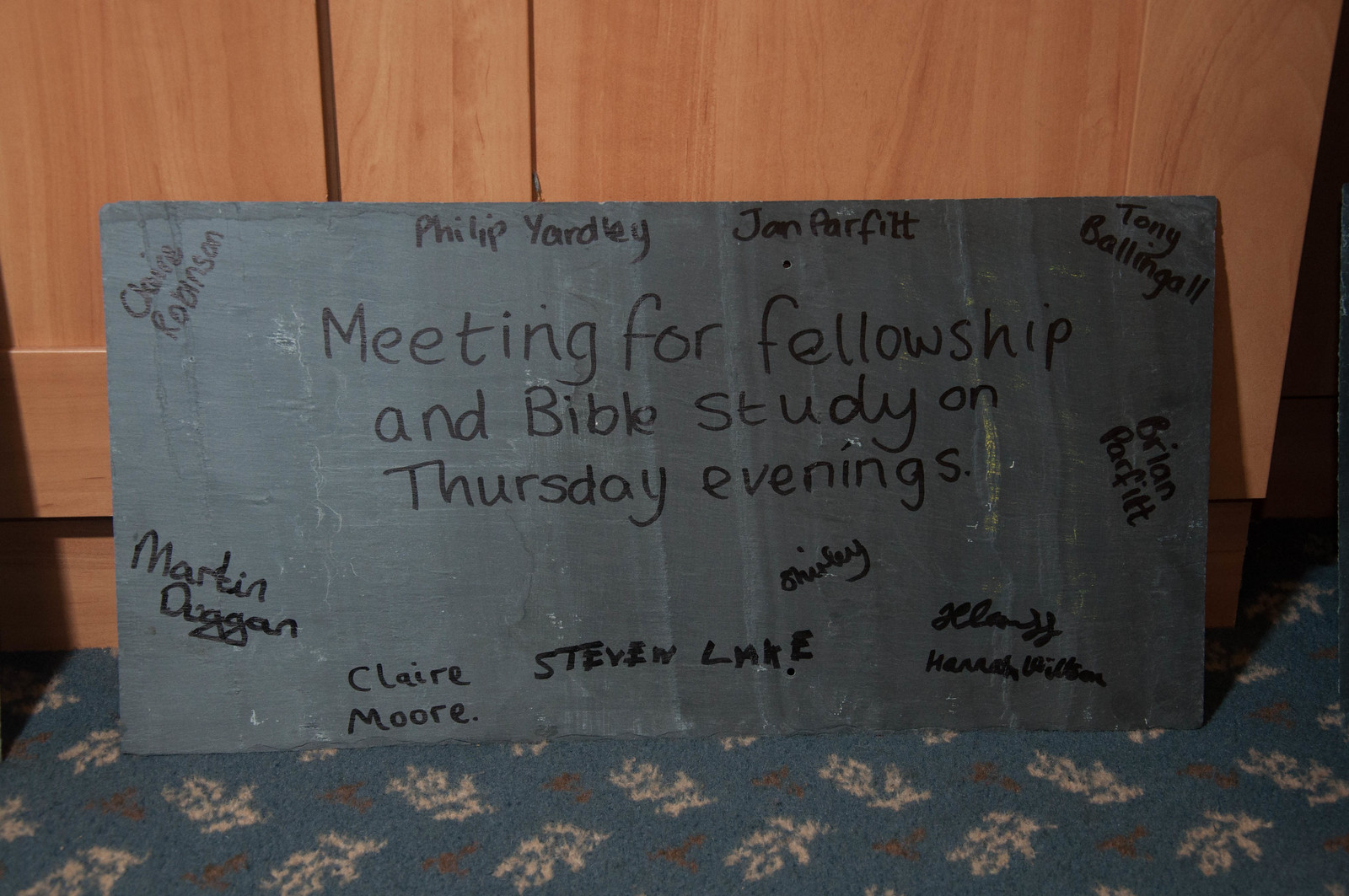The photograph showcases a dark gray homemade sign, approximately rectangular in shape, leaning against a wooden cabinet. The sign is placed on a blue carpet with white and gray patterns. The sign, likely made from creased poster board, prominently displays the message "Meeting for Fellowship and Bible Study on Thursday evenings" centered in black text. Surrounding this central message are various names written or signed in black, positioned around the edges of the sign. Starting from the upper left corner, the names include Claire Robinson. Moving to the right of her name is Philip Yardley, followed by Jan Parfit and Tony Bellingall in the upper right corner. Below Tony’s name is Britton Parfit. Continuing to the bottom right corner, the names listed are Hilary Hilton and Shirley. Moving left from there, Stephen Lake and Claire Moore are named, with Martin Dagen’s signature situated in the bottom left corner.